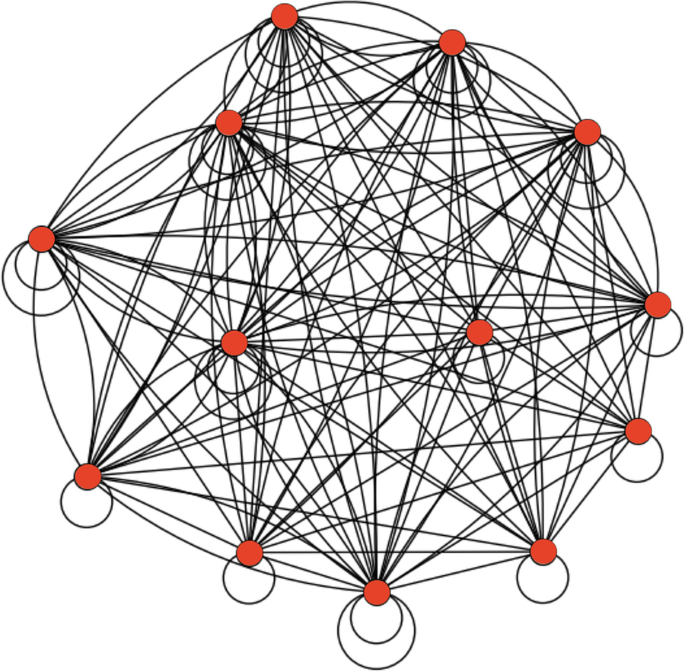The image features a hand-drawn or possibly computer-generated diagram with 13 to 15 red circles distributed unevenly in a generally circular pattern against a white background. Each red circle has either one or two black outline circles emanating from it; those on the bottom typically have one outline while those on top and to the left mostly have two. These red circles are interconnected by numerous black lines, creating a complex, web-like structure that gives the diagram a mandala-like, hypnotic appearance. The dense network of lines crisscrosses the image, making it resemble a chaotic, yet oddly geometric pattern. The overall effect is intricate and mesmerizing, though the exact purpose or representation of the diagram remains unclear.